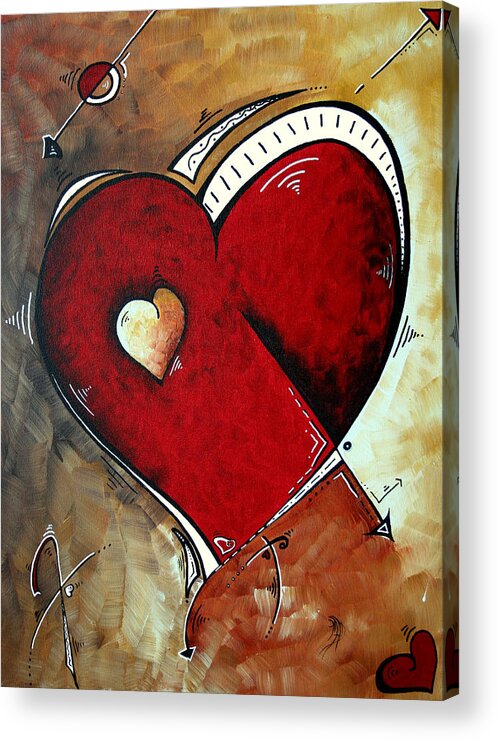The painting depicted is a modern, stylized artwork presented on a canvas, encompassing a predominant red heart centered in the composition. Within this main heart lies a smaller, brown and white heart, adding a layered dimension to the piece. The background is marked by a goldish-beige hue with shimmering accents of brown, white, red, and subtle gray lines. Multiple arrows and lines intersect the composition at varied angles, with notable features including a red arrow in the upper right corner and an orange, white, and red circular arrow. A smaller dark red heart occupies the bottom right corner, encircled by a white outline, while a signature or letter "F" appears in the bottom left. The painting extends over the edges of the canvas, eliminating the need for a frame and giving a sense of continuity. The overall impression is of an amateurish yet vibrant modern art piece, rich with random squiggles and dotted lines, possibly showcased as a stock image.